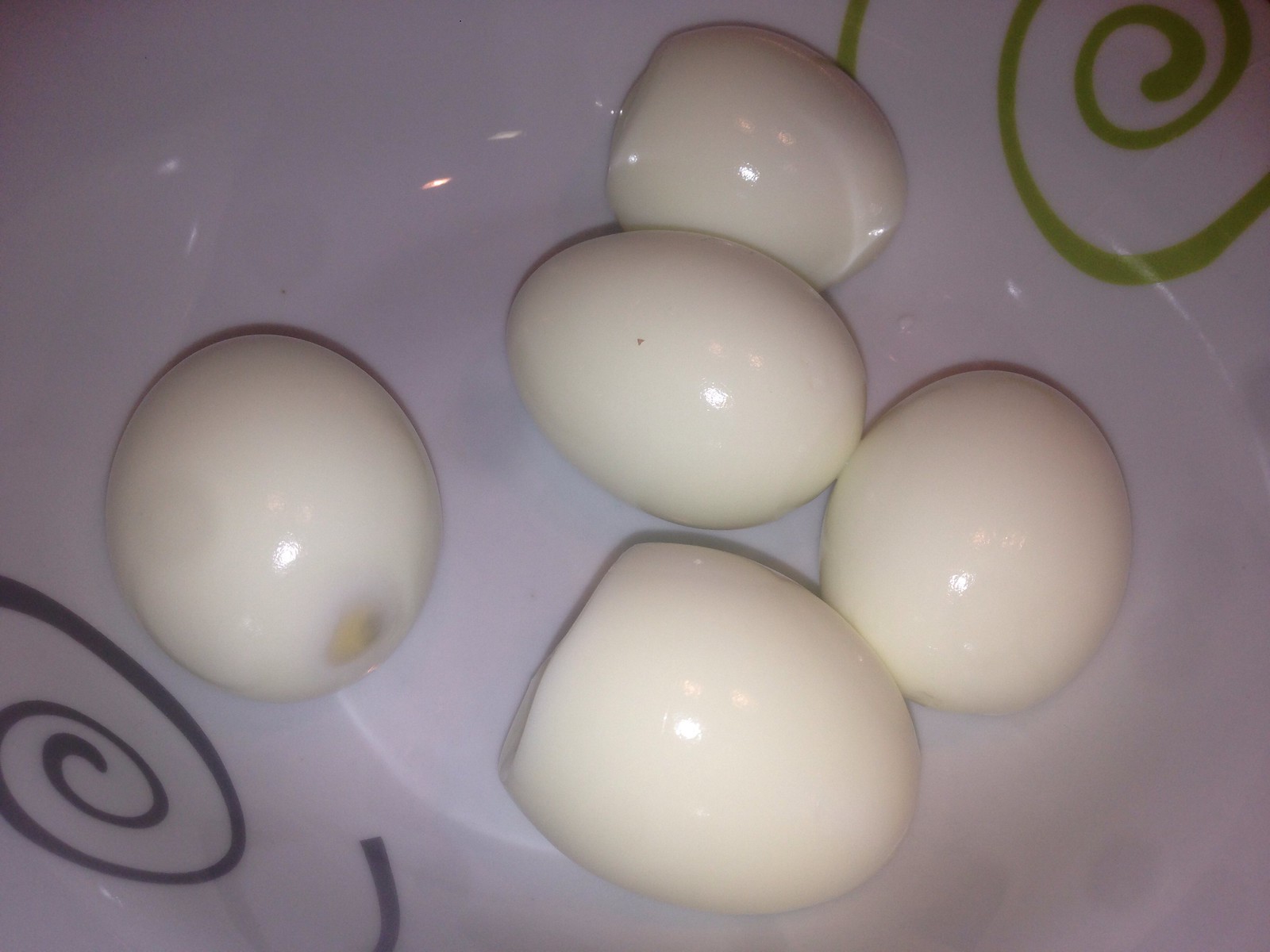This indoor color photograph captures a close-up of five peeled hard-boiled eggs arranged in a ceramic bowl or on a platter. The image is taken from above, and the edges of the dish extend beyond the frame on all sides. The dish is off-white with decorative squiggly designs: a prominent black squiggle in the bottom left corner and a light green spiral in the top right corner. The five eggs are organized with four of them touching each other in the center; three eggs form a central column, one egg touches this column on the right, and another egg sits alone on the left side of the photo. Notably, this left egg has a small bit of yolk peeking out on its far side. The light source above creates a slight reflection on the smooth surfaces of the eggs, emphasizing their glossy texture. No text or markings are visible in the photograph.